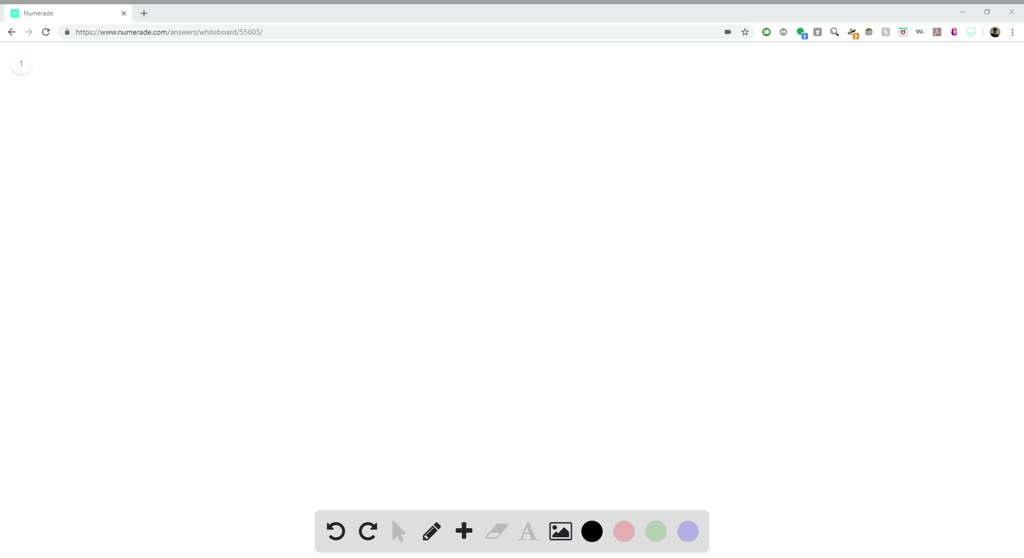This image appears to be a screenshot of a desktop interface, possibly from a drawing application, but the screen itself is blank. At the top, there is an open folder with a small blue icon beside an illegible name, an 'X' button for closing the folder, and a plus sign. On the far right, another 'X' button is visible to close the entire window. 

On the left side below the folder icon, a highlighted arrow pointing left is present, with a faded arrow pointing right next to it, followed by a circled arrow. Adjacent to these is a search bar that ends with a star icon and what seems to be a camera icon, along with various other icons further to the right.

At the bottom of the screen, a toolbar is clearly visible. This toolbar includes a redo arrow, a forward arrow, an upward arrow, a pencil icon, a plus sign, an eraser, the letter 'A,' an image icon, and several colored dots, presumably for selecting different colors.